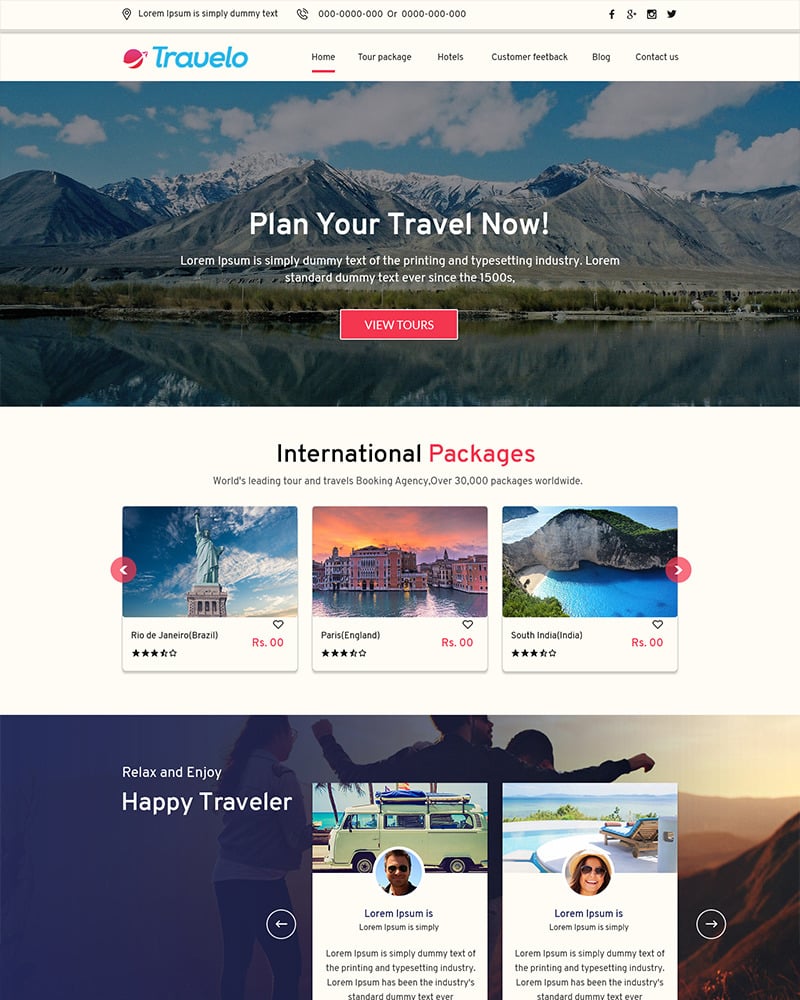The header section of the website begins with a grey strip running across the top-left, where the words "Laurium Ipusum" – simple dummy text – are displayed. Adjacent to this text is a placeholder phone number composed entirely of zeros. On the right side of the grey strip, social media icons for Facebook, Google+, Instagram, and Twitter are prominently placed.

Beneath this strip is another thin grey line, under which the brand name “Travelo” is showcased in blue. Adjacent to "Travelo," there is a dynamic red circle with a white arrow curving around it from the left and pointing outward. To the right of this logo, there is a neatly organized navigation bar with the following menu items: Home, Tour Package, Hotels, Customer Feedback, Blog, and Contact Us. The "Home" menu item is underlined in red, indicating the current page, while the other menu items are styled in black against a white background.

Below the navigation bar, a stunning photograph of snow-capped mountains under a clear blue sky captures attention. A serene lake lies in the foreground, perfectly mirroring the majestic mountains. Overlaid centrally on the image is the motivational text "Plan Your Travel Now." Beneath this text, a block of traditional dummy text provides a placeholder narrative about the printing and typesetting industry. Additionally, a prominent red button with the text “View Tours” invites users to explore further. The content below this section continues on a clean white background.